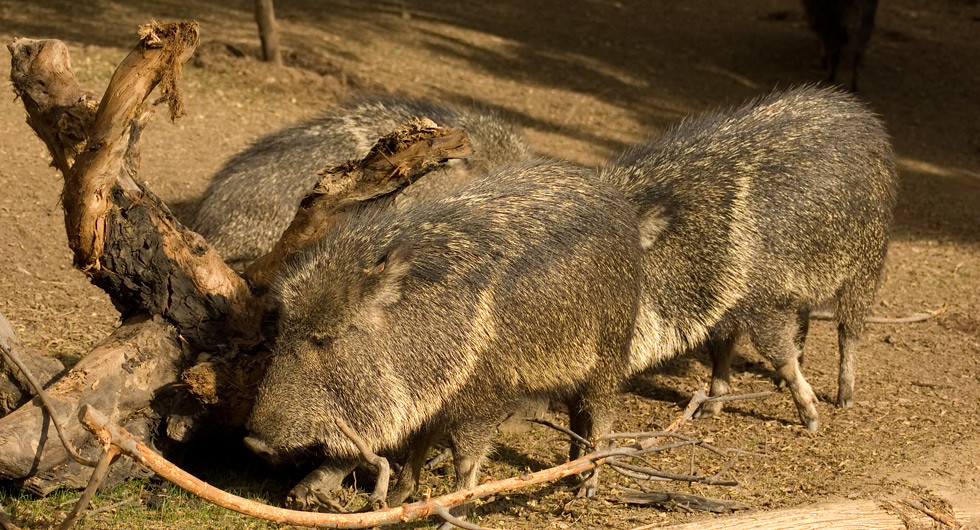The image captures a close-up, horizontal, rectangular shot of three small, furry animals likely located in a zoo setting. The ground beneath them is a dusty, tan-brown sandy dirt, scattered with what appears to be wood pulp. Prominent on the ground are numerous wooden logs, some possibly cut in half, suggesting the animals might use these for chewing or play.

The animals resemble a blend between pigs and capybaras, possessing distinct features from both. They have short, sturdy bodies with big heads that are almost equal in size to their bodies. Each animal stands on four legs, ending in what look like little hooves. Their fur appears quite spiky and rough to the touch, a mix of grayish-brown, black, beige, and dull yellow hues. The texture of their fur is more rigid than soft, and spines or porcupine-like quills are noticeably absent.

Their faces are marked by dark eyes and protruding snouts, giving them a distinctive appearance. Additionally, two ears are visible atop each head. These animals are grouped closely together, standing near a large bare branch on the ground, which adds to the rustic and barren ambiance of their desert-like environment.